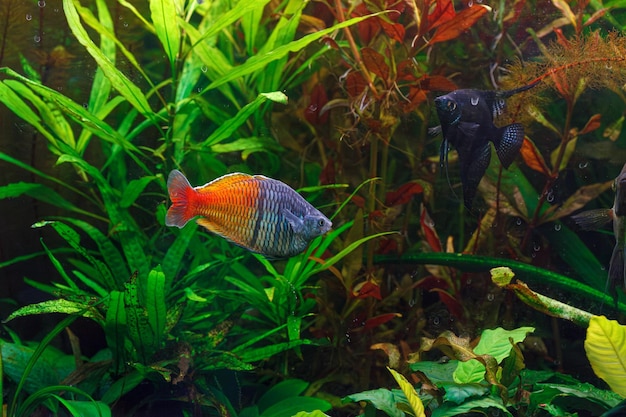The image portrays a detailed scene in an aquarium, highlighting a singular fish at the center. This fish is vividly multicolored, featuring an orange tail and a blue head, giving it a striking appearance. Its scales appear to blend between orange and blue, adding to its unique beauty. The aquarium itself is spacious, adorned with a variety of plants; a lush greenery dominates the background while reddish vegetation can be seen to the right. The environment is well-lit, with light streaming down from the top of the image. A second fish, darker and more triangular in shape with prominent fins, swims from the right edge towards the upper right-hand corner. This fish contrasts sharply with the more oval-shaped, colorful fish at the center. Despite having only two fish, the aquarium looks vibrant and dynamic with its mix of green and orange vegetation, and an overall ambiance that is slightly murky yet lively.